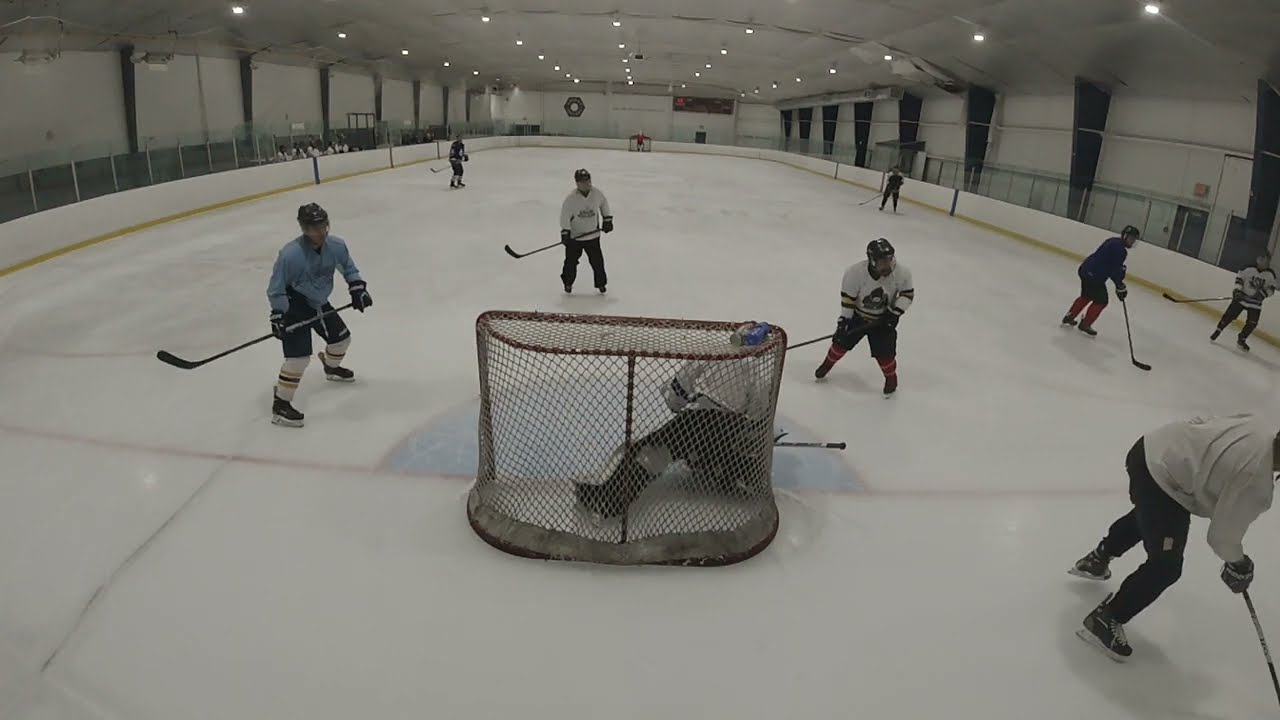This image captures an intense moment in a hockey rink from the perspective of a spectator behind the goalie. At the focal point, the goalie is seen crouched down on the ice, with one foot inside the goal and his stick extended to his right. Directly in front of him is a player, flanked by two others on his left and right, all with their hockey sticks angled to the left. In the bottom right of the image, a player in a white shirt and black pants holds his stick down towards the ice. Above him to the right, a player in a dark uniform, black helmet, and red pants sets his stick on the ground. Alongside him, another player at the edge of the rink, dressed in a white jersey, also positions his stick towards the left. In the background, two players in dark jerseys have their sticks pointed downward towards the play. The rink is encircled by a white barrier, beyond which a chain link fence is visible. The ceiling features a row of lit lights stretching from front to back. The ice in front of the goalie is marked with light blue and red lines. The scene, devoid of a crowd, suggests a practice session rather than an actual game.